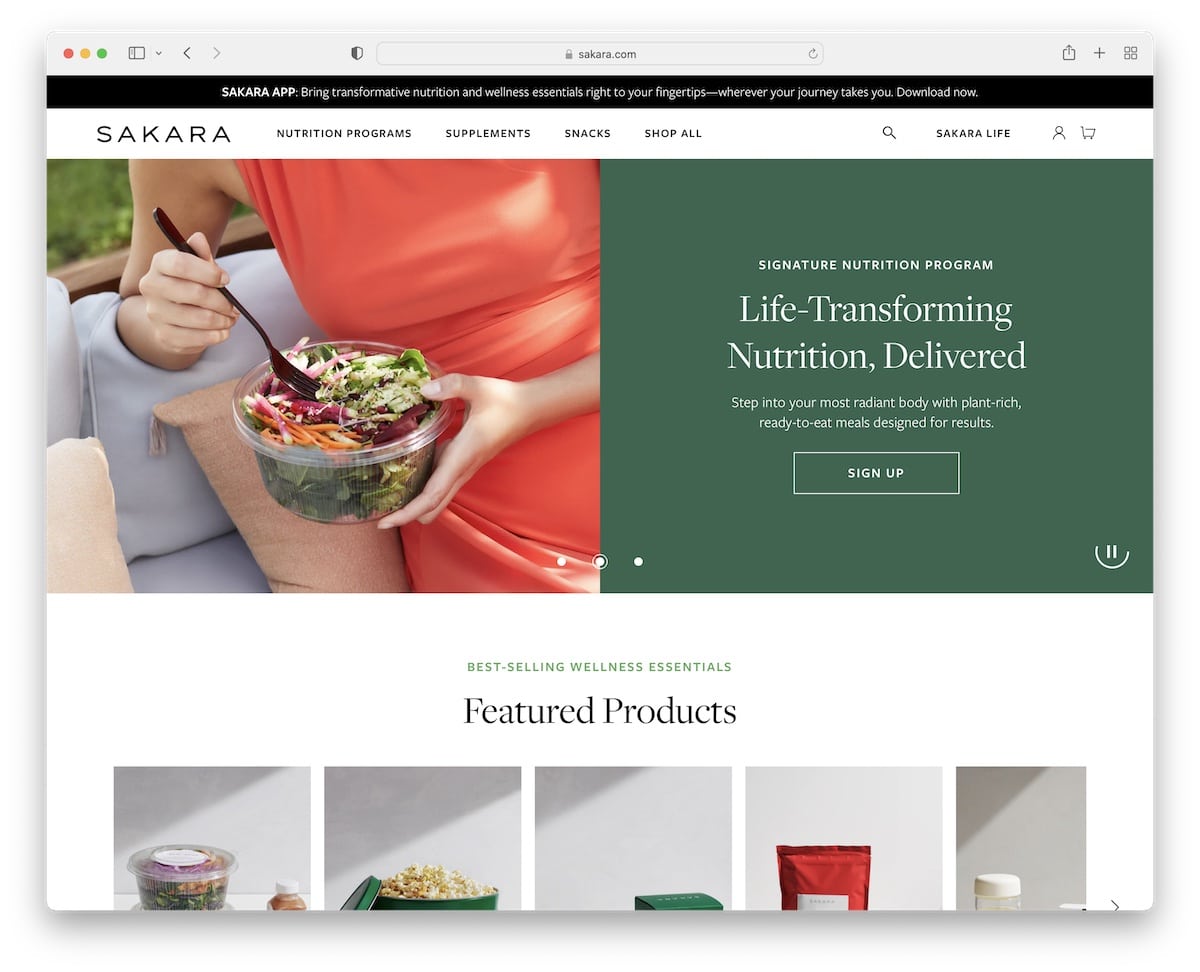The image displays an appealing website layout for Sakara, an online platform specializing in transformative nutrition and wellness. At the top, a black banner states: "Sakara app: Bringing transformative nutrition and wellness essentials right to your fingertips wherever your journey takes you. Download now." Below the banner, the site's menu features options such as "Nutrition Programs," "Supplements," "Snacks," and "Shop All," with a magnifying glass icon for search functionality to the right. "Sakara Life" is prominently displayed next to a small profile icon and a shopping cart.

The primary image showcases a woman in a red dress lounging outdoors, enjoying a vibrant salad filled with colorful ingredients like beets, carrots, and cucumbers. To the image's right, text reads: "Signature Nutrition Program: Life-transforming nutrition delivered. Step into your most radiant body with plant-rich, ready-to-eat meals designed for results. Sign Up."

Below, the section titled "Best-Selling Wellness Essentials" introduces featured products displayed in a row of five squares. The first square appears to contain the same salad enjoyed by the woman. The second square looks like it holds popcorn. The third is a nondescript blue box, while the fourth contains a red bag. The fifth square shows the top of what could be a container or shaker bottle.